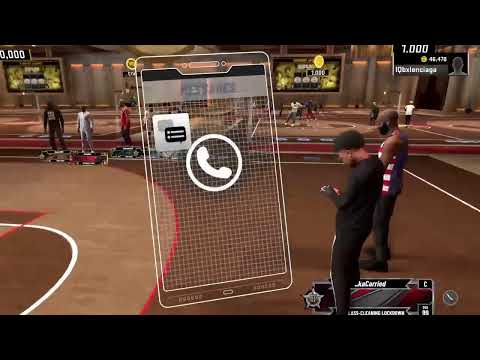The image features a screenshot from a video game, set against a black background at the top and bottom. Prominently displayed is the graphic of a rectangular, vertically-oriented mobile or tablet device. This device has a distinctive round white button at the bottom, marked with a telephone handset icon and a white grid-like pattern.

Behind the mobile device graphic, the scene showcases a virtual basketball court, characterized by a predominantly brown surface with red and white accents. Several in-game players are visible on the court, immersed in the action. Surrounding the court are screens displaying scores and graphics, including a highlighted number at the top, "7,048,476," presumably indicating the current game score or points.

To the right of the court, two characters are prominently positioned. One character wears a colorful basketball jersey in red, white, and blue, paired with short sleeves. Next to him stands another character dressed in a black long-sleeved shirt and black pants, contrasting sharply with the vibrant athletic attire of his companion. The overall scene captures the dynamic environment of a basketball game within the video game, blending elements of virtual sports and user interface design.